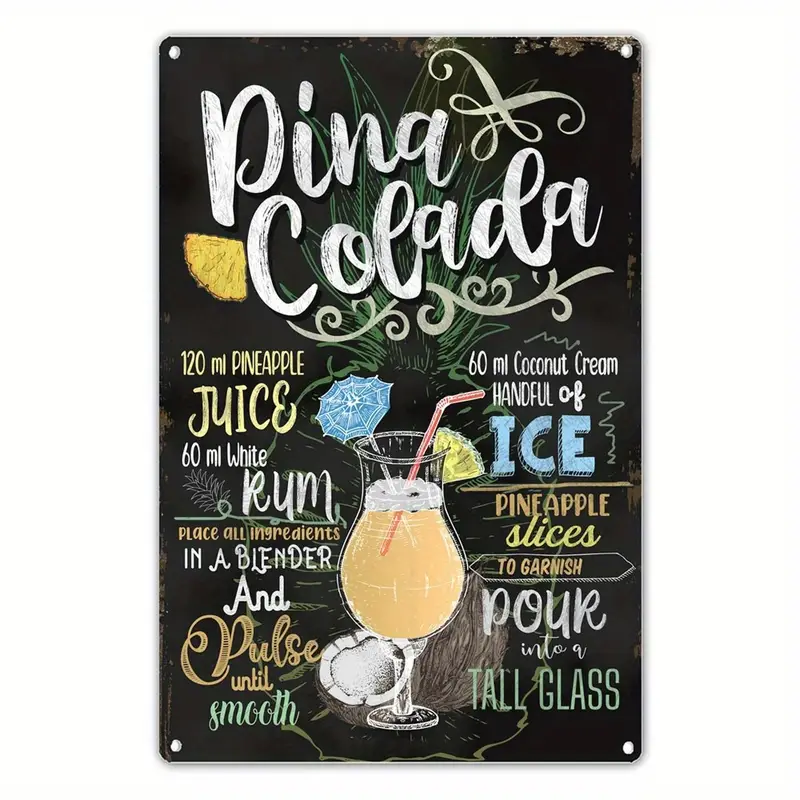This image displays a charming sign reminiscent of those you'd find outside a quaint cafe or bar, advertising a piña colada. The background of the sign is black, providing a striking contrast to the vibrant elements. At the top, the words “Piña Colada” are written in large, elegant white script, flanked by a slice of pineapple near the letters 'P' and 'C'. Faintly encircling the piña colada recipe is the green, sketched outline of a whole pineapple, blending into the background. 

Below the title, the sign features a detailed recipe for making a piña colada. Centrally positioned in the lower part of the sign is a tall, stemmed glass filled with the tropical drink, colored a vibrant orange. The glass is adorned with a bendy straw, a blue cocktail umbrella, and a slice of pineapple on the rim. An open coconut behind the glass adds to the tropical aesthetic. 

The recipe reads: "120 milliliters pineapple juice, 60 milliliters white rum. Place all ingredients in a blender and pulse until smooth." On the right-hand side, additional instructions add: "60 milliliters coconut cream, a handful of ice, pineapple slices to garnish. Pour into a tall glass."

The subtle details, such as the split coconut and the background greenery, further enhance the inviting, tropical ambiance of the sign, making it a perfect decorative piece for a cafe or kitchen setting.